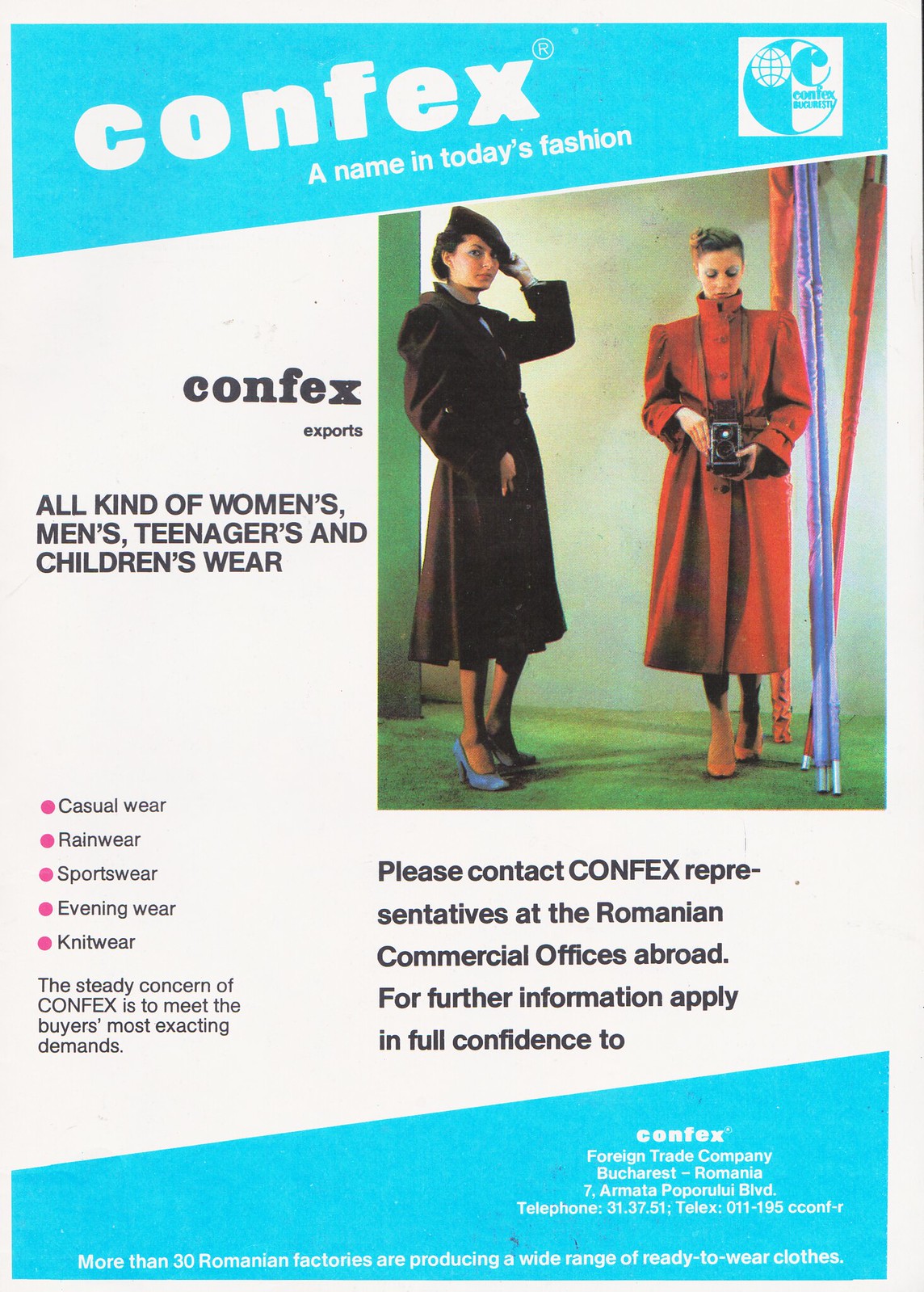This print advertisement features a striking image set against a white background, framed with turquoise banners at the top and bottom, each containing white text. The top banner showcases the headline, "Confex, a name in today's fashion," alongside a logo resembling a globe intersected by a 'C'. Centrally positioned, a photograph captures two women in model-like stances, each adorned in heavy peacoats—one in brown and the other in black, with the woman on the right holding an old-fashioned camera. The ad likely hails from the 60s or 70s, given the fashion style and camera design. 

The explanatory text below the image emphasizes, "Confex exports all kinds of women's, men's, teenagers' and children's wear," and invites the reader to "please contact Confex representatives at the Romanian commercial offices abroad." Additional details in the bottom turquoise banner provide contact information, including an address, telephone, and telex number in Bucharest, Romania, noting that more than 30 Romanian factories are producing a wide range of ready-to-wear clothing.